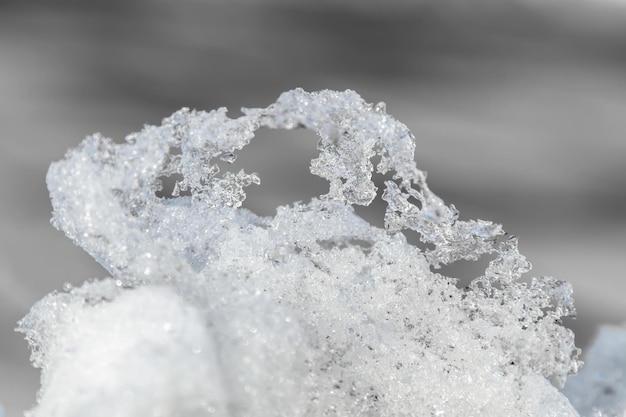A close-up of an icicle, possibly a frozen leaf or flower, dominates the scene. The ice is pristine and crystalline, emerging thick from the bottom and tapering delicately to the top, almost forming holes as it becomes less dense. The colors of the ice range from white and gray to hints of blue, giving it a diamond-like appearance. This icy structure is set against a fuzzy, blurred background of gray and white shades, enhancing the purity and texture of the ice. The image, wider than it is tall, conveys a sense of icy stillness with scattered, dirty ice chunks and a touch of black debris, hinting at the melting process. The contrast between the sharp detail of the ice and the soft, cloudy background makes the icicle stand out strikingly.